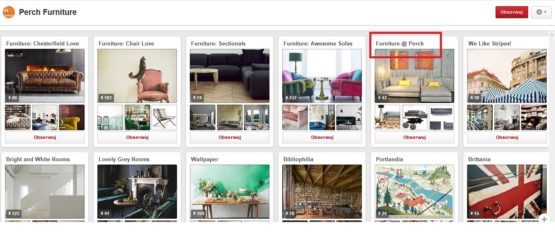This image showcases the Perch Furniture website, structured into a 6x2 grid displaying 12 colorful photos of various furniture items. The top row contains six detailed images, each prominently featuring a specific furniture piece. Below each of these primary photos, three smaller images display similar or related items, providing a comprehensive view of the product range.

The bottom row of the grid also contains six images but differs from the top by solely displaying the main pictures without the additional thumbnails. The captions for these images include: "Furniture Chesterfield Love," and "Furniture Chair Love." The remaining descriptions for the top images relate to different types of furniture pieces.

For the bottom row, the captions are diverse, highlighting themed rooms and other categories: "Bright and White Rooms," "Lovely Gray Rooms," "Wallpaper," (an unreadable caption), "Post Media," and "Britannia." This layout gives a succinct yet thorough glimpse into the diverse offerings and thematic collections available on the Perch Furniture site.